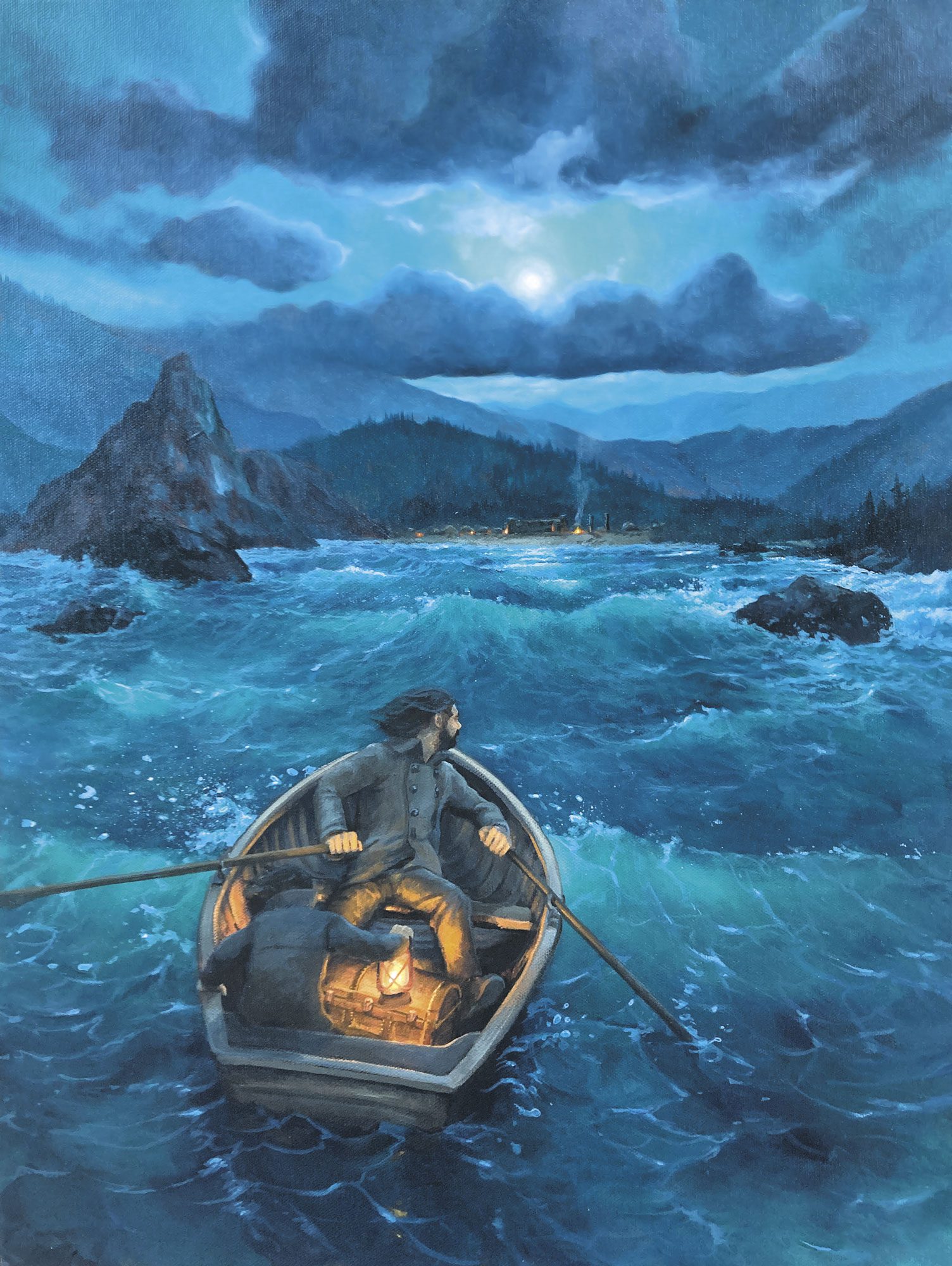The image features a detailed illustration of two men struggling in a small, brown rowing boat amidst a stormy sea. The man at the oars, casting a fearful glance over his shoulder, seems to be checking their precarious situation, possibly fearing pursuit or the treacherous waves. Positioned at the back of the boat, the second man holds a bright yellow lantern glowing with a warm orange light, providing stark contrast to the turbulent surroundings. The sea beneath them is a swirling mix of dark and light blues, with foam-tipped waves crashing violently. Jagged boulders punctuate the water surface, adding to the sense of danger. To the left, a tall cliff rises abruptly from the sea. In the distant background, faint fires burn on the land, their smoke curling upwards, hinting at a hasty escape by the men. These distant fires are set against a landscape of imposing mountains, some covered in trees while others remain barren and rocky. Above, dark ominous clouds roll through a blue sky, partially obscuring the sun or perhaps the moon, as the men row desperately towards the shore. The entire scene, painted with a sense of looming peril, encapsulates the raw power of nature and the men’s struggle for survival.